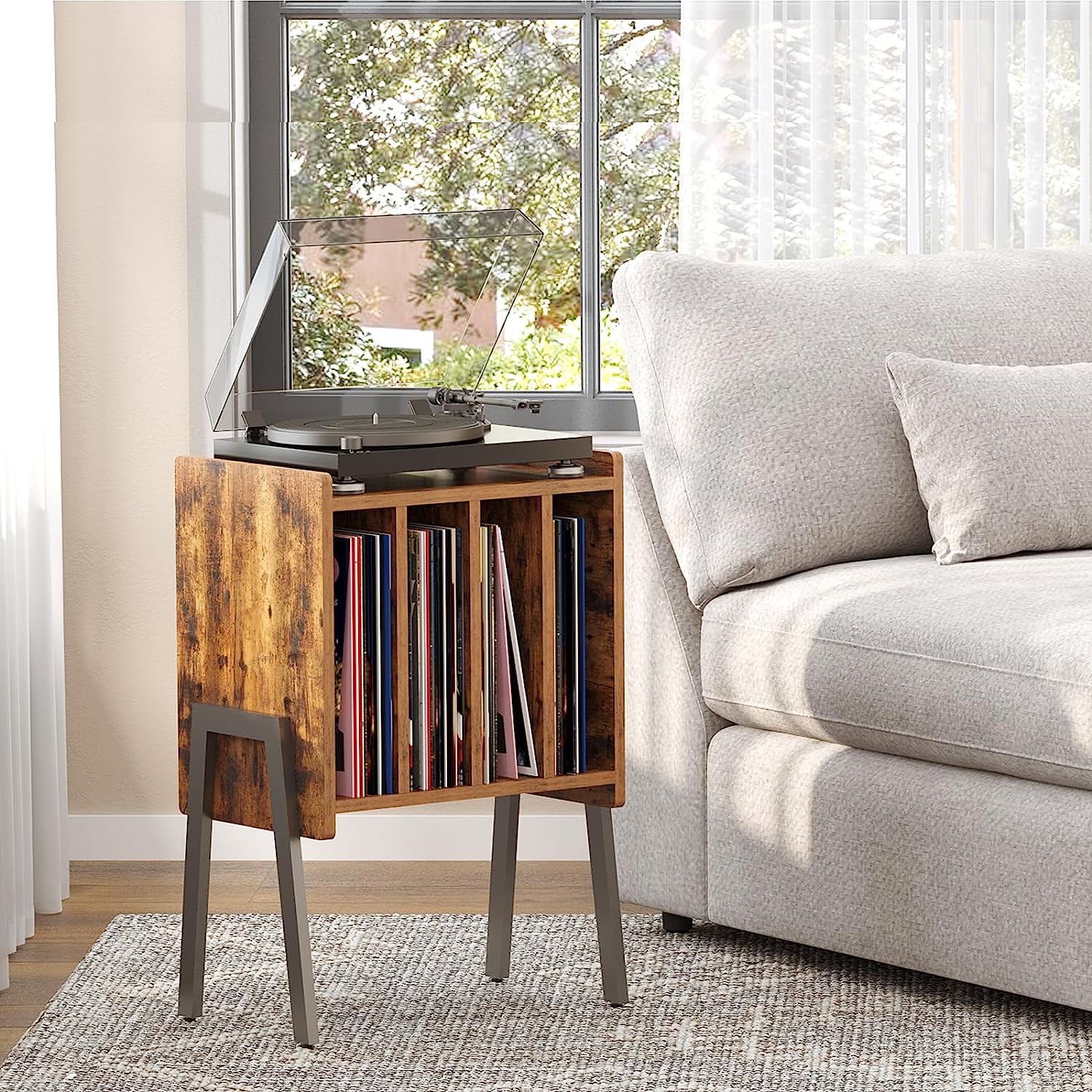The image depicts a meticulously staged and clean interior, likely a living room, showcasing a stylish setup centered around a vinyl record collection. The focal point is a wooden album holder, crafted from a brown burnt wood-like material, with gray metal legs supporting it on either side. The front of the holder features four cubbies, each filled with vinyl records. Atop this piece of furniture sits a modern plastic spin turntable, its clear plastic lid currently open, revealing a record inside. 

The room itself has white painted walls with multi-pane windows framed in gray. Sheer white curtains partially cover the windows, through which natural sunlight filters into the room, casting a soft glow on the scene. A gray fabric-covered couch is visible to the right of the record holder, adding to the cozy yet contemporary ambiance. The floor is wooden, accented by a gray and white rug that sits beneath the album holder and turntable stand. The setting is further enriched by the presence of greenery visible outside the window, contributing to the serene and inviting atmosphere of the space.